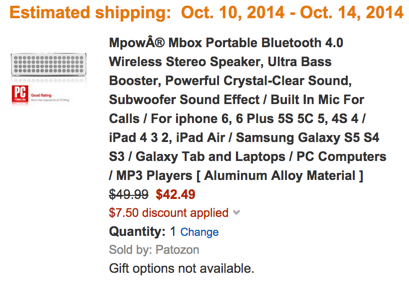This image features a screenshot set against a pristine white background. At the top, bold orange text prominently displays the estimated shipping dates: "October 10, 2014 through October 14, 2014." Below, in bold black text, there's an extensive product title: "MPOWA M-Box Portable Bluetooth 4.0 Wireless Stereo Speaker Ultra Bass Booster Powerful Crystal Clear Sound Subwoofer Sound Effect Built-in Mic for Calls For iPhone 6, 6 Plus, 5S, 5C, 5, 4S, 4, iPad 4, 3, 2, iPad Air, Samsung Galaxy." In striking red text beneath this description, the price is shown as "$42.49" with a "$7.50 discount applied." The product is sold by "PatoZone."